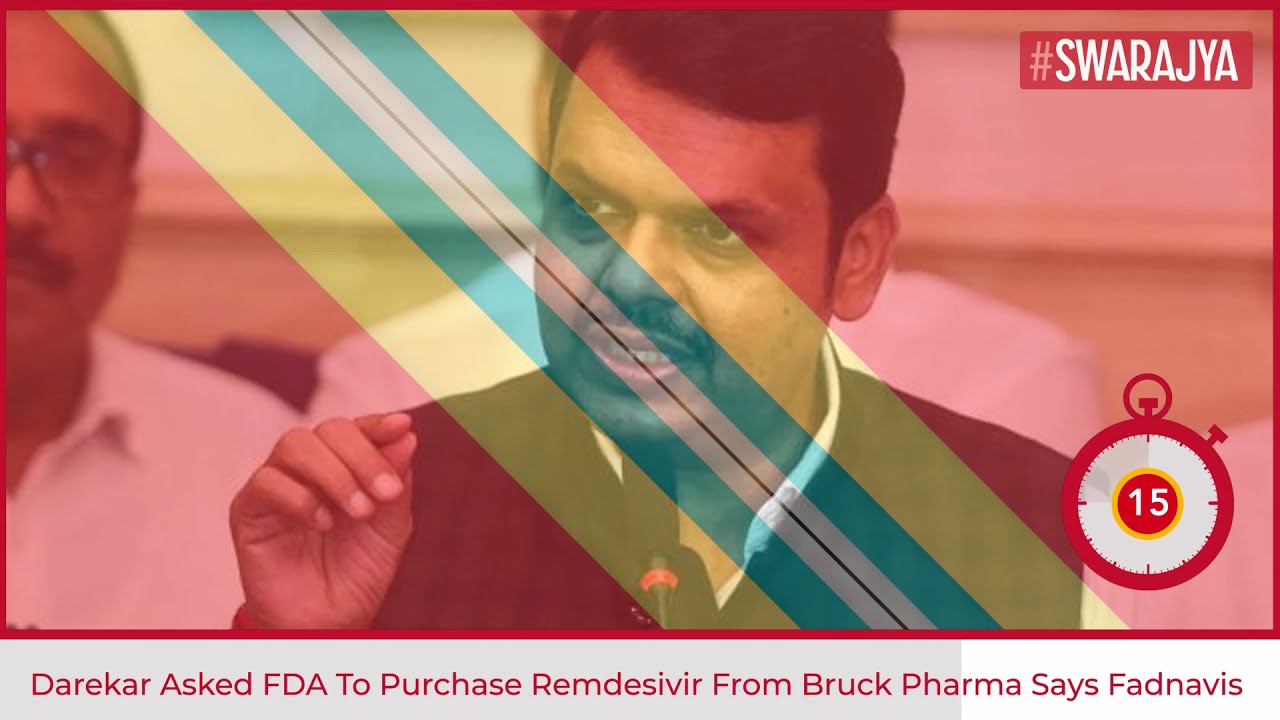The image appears to be a screenshot from a TV broadcast or an article, characterized by a distinct, dark red rectangular border and an overall reddish tint. Across the top right-hand corner is a dark red horizontal rectangle displaying the hashtag "SWARAJYA" in white uppercase letters. In the bottom right-hand corner, there is a red stopwatch icon with the number "15" prominently displayed in the center in white font.

The central figure in the image is a dark-skinned man of possible Middle Eastern or Indian descent, wearing a black suit jacket and a white shirt. He has short black hair, a mustache, and pronounced bags under his eyes, suggesting a weary appearance. He is speaking into a thin microphone, his right hand extended outward, and his expression conveys anger or intensity. A second man, described as possibly bald with glasses and a mustache, can be seen in the background, looking toward the speaker.

Across the image, there is a pattern of soft pastel stripes running diagonally from the upper left to the lower right, consisting of yellow, blue, gray, and a thin black stripe. Additionally, there are broader bands of yellow and blue with inner white stripes, possibly evoking a flag or similar design.

Beneath the image lies a gray rectangular banner featuring dark red text that reads: "Derrick Carr asked FDA to purchase remdesivir from Brook Pharma, says Fadnavis."